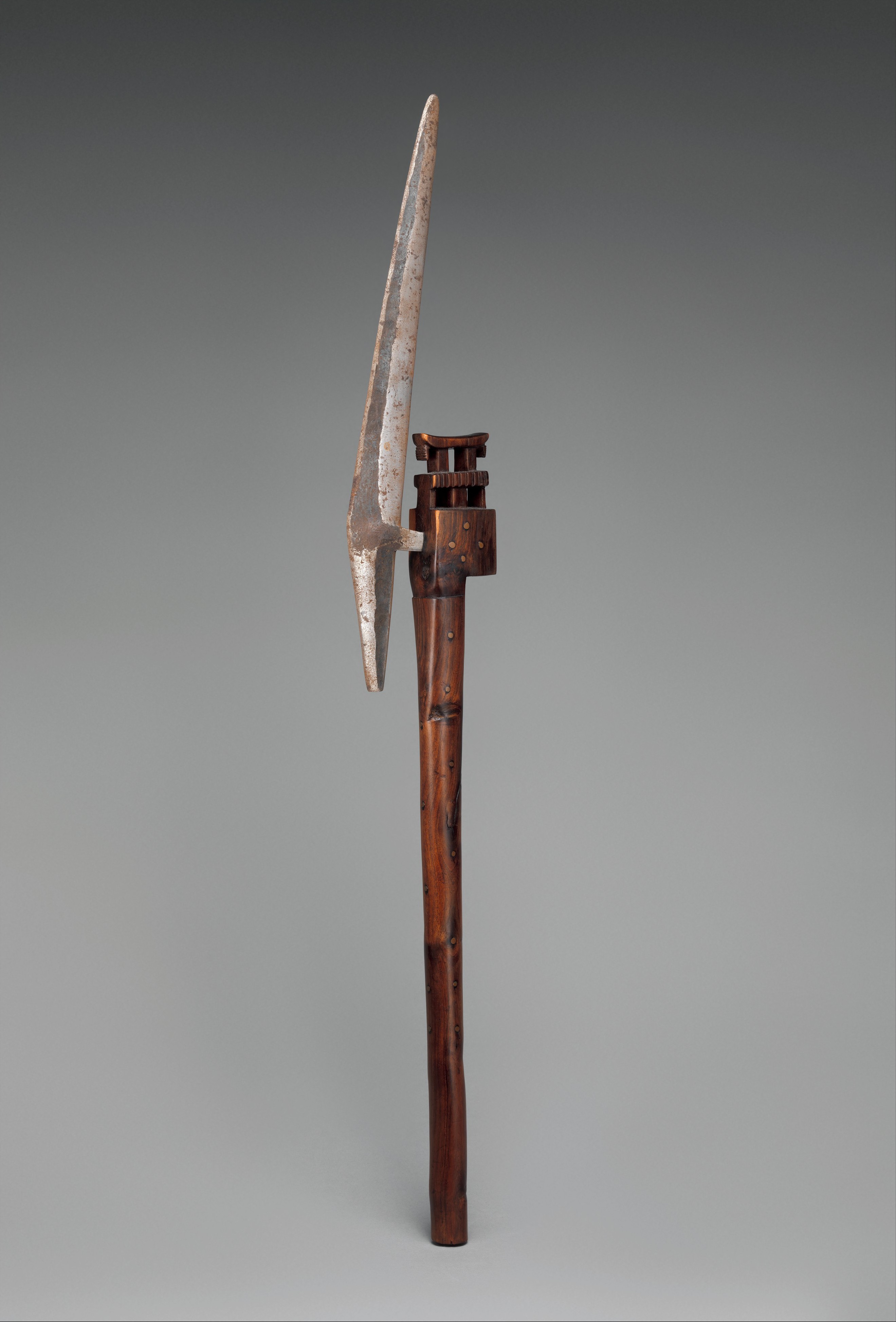The image features a prominently displayed object, possibly a tool or weapon, standing upright against a solid gray backdrop. The object consists of a brown wood-colored or bronze handle with some black shadings, described as a long cylindrical pole. Attached to the top of the pole is a square-shaped block with intricate design work that secures a silvery, steel blade. The blade, shaped like a long triangle with sharp edges, shows signs of rust with brown markings. The background is a gradient, darker gray at the top and lighter gray at the bottom, providing a neutral, textureless setting that makes the object the focal point of the image.